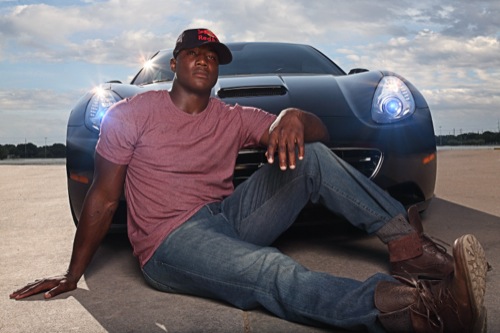The photograph captures a man centered in the image, sitting on the ground in front of a sleek, low black sports car with a silver grill. The car faces forward in a large gray asphalt parking lot. The man, slightly angled to the right but facing forward, supports himself with his right hand on the ground and rests his left forearm on his bent left knee. His right leg extends straight to the right, while his left leg and knee create a bend. He is dressed in blue jeans, brown leather boots, and a short-sleeve purple (or dark pink) t-shirt. He dons a black baseball cap with a see-through mesh side and a red logo on the front. Behind him, the sky occupies half of the image, showcasing a light blue backdrop filled with contrasting white and dark gray clouds. Flanking the scene in the distance, a tree line of lush, green-leaved trees adds depth to the composition.